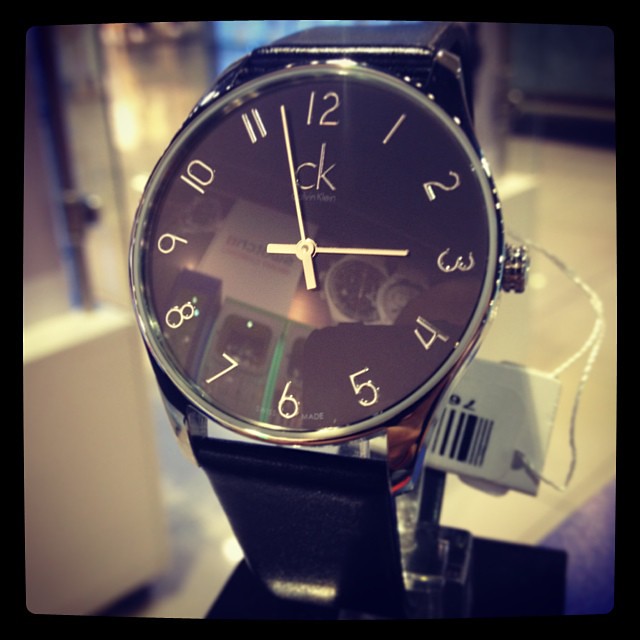A square image featuring a somewhat blurry depiction of a watch centrally placed. The watch has a black band and a circular face with a black background. White numbers are clearly visible, and a silver knob is present on the right side of the watch face. In the blurred background, there are indistinct items, with a specific white tag noticeable behind the watch on the right side. Despite the low image quality, the key details of the watch are discernible.